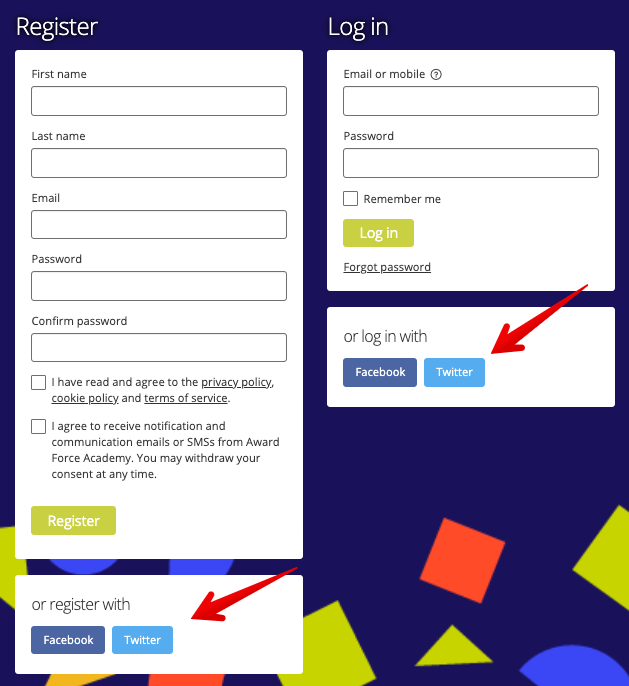This image depicts a website's user interface for registration and login, set against a blue background and presented in a portrait layout, approximately one and a half times taller than it is wide. 

On the left side, there is a registration section titled "Register" in white lettering. Below this title, there is a vertical, portrait-style form with a white background, containing five input fields labeled: First Name, Last Name, Email, Password, and Confirm Password. Beneath these fields, there are two checkboxes. The first checkbox allows users to indicate that they have read and agreed to the privacy policy, cookie policy, and terms of service. The second checkbox grants permission to receive notifications and communication emails/SMS from AwardForce Academy, with a note stating that consent can be withdrawn at any time. At the bottom of this form, there is a greenish-yellow "Register" button with white text. Below the button, an additional option to register via social media is provided, featuring a smaller, landscape-oriented white box with the text "Or register with." This box includes blue Facebook and blue Twitter buttons, with Facebook being a darker blue and Twitter a lighter blue, both featuring white text. A red arrow points to the Twitter button.

On the right side, the login section is titled "Login," also in white lettering. This section features two input fields: one for Email or Mobile and one for Password. Below these fields, there is a checkbox labeled "Remember me," and a green "Login" button. Additionally, there is a "Forgot Password?" link below the login button. Similar to the registration form, this section includes the same options to log in via Facebook and Twitter, presented as blue buttons with white text.